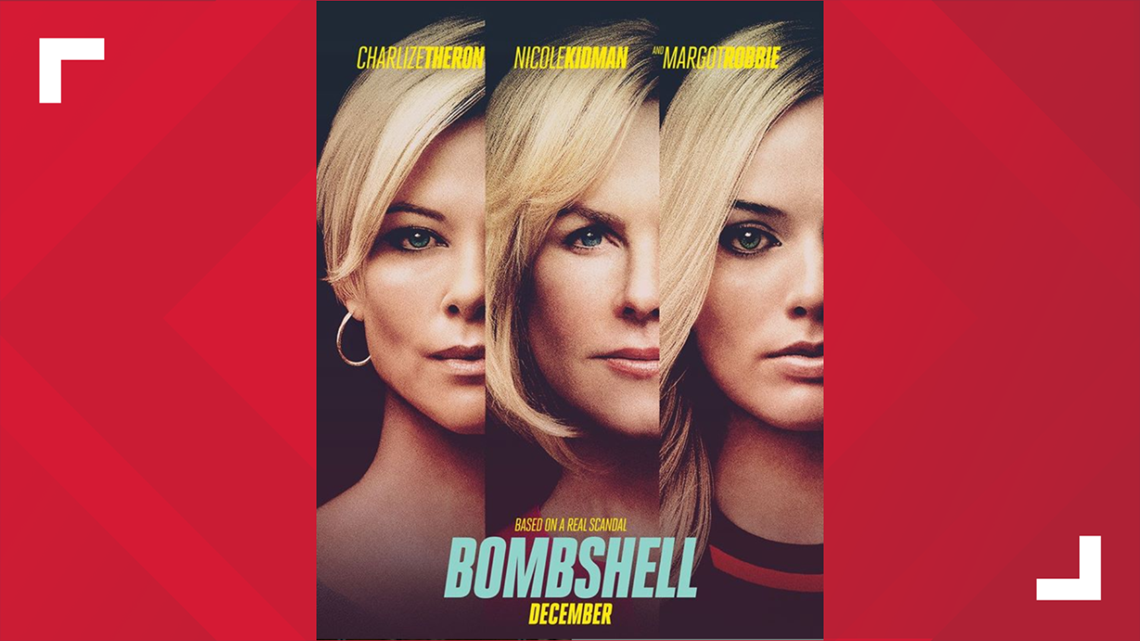This detailed movie poster for "Bombshell" features three prominent blonde actresses—Charlize Theron, Nicole Kidman, and Margot Robbie. Each woman's headshot is cut in half and overlaid side by side, showcasing just one side of their faces in a compelling alignment. Above each face, their names are written in striking yellow font. 

The poster's background is defined by distinctive red borders with geometric triangle patterns suggesting motion, along with small white L-shaped markings in the corners. At the top, it states that the movie is "Based on a Real Scandal," emphasizing the dramatic nature of the film. The title "Bombshell" is boldly written in light blue capital letters, with the release month "December" prominently displayed in yellow beneath it.

Each actress is slightly smiling with their hair swept to the side, highlighting their blue eyes and dark shirts that add to the poster's intense aesthetic. Notably, Charlize Theron, wearing short hair and visible earrings, stands out as the other women have medium to long hair, potentially covering any jewelry. The unified expression of the actresses, coupled with the vibrant color scheme, makes the poster both eye-catching and memorable.